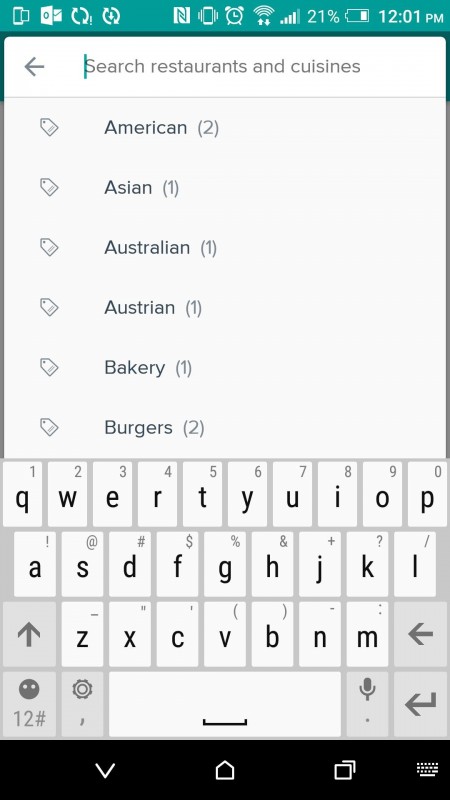This image is a screenshot from a mobile device, showcasing a user interface with a green status bar at the top. The status bar includes several notification icons. Below this, there is a navigation arrow pointing to the left, adjacent to a search bar with the placeholder text "Search restaurants and cuisines." Within the search bar, there's a drop-down list of suggested search filters, each accompanied by a gray tag icon. The suggestions start with "American" (2 results), followed by "Asian" (1 result), "Australian" (1 result), "Austrian" (1 result), "Bakery" (1 result), and "Burgers" (2 results). Beneath this suggestion list, the on-screen keyboard is visible, featuring a light gray color scheme.